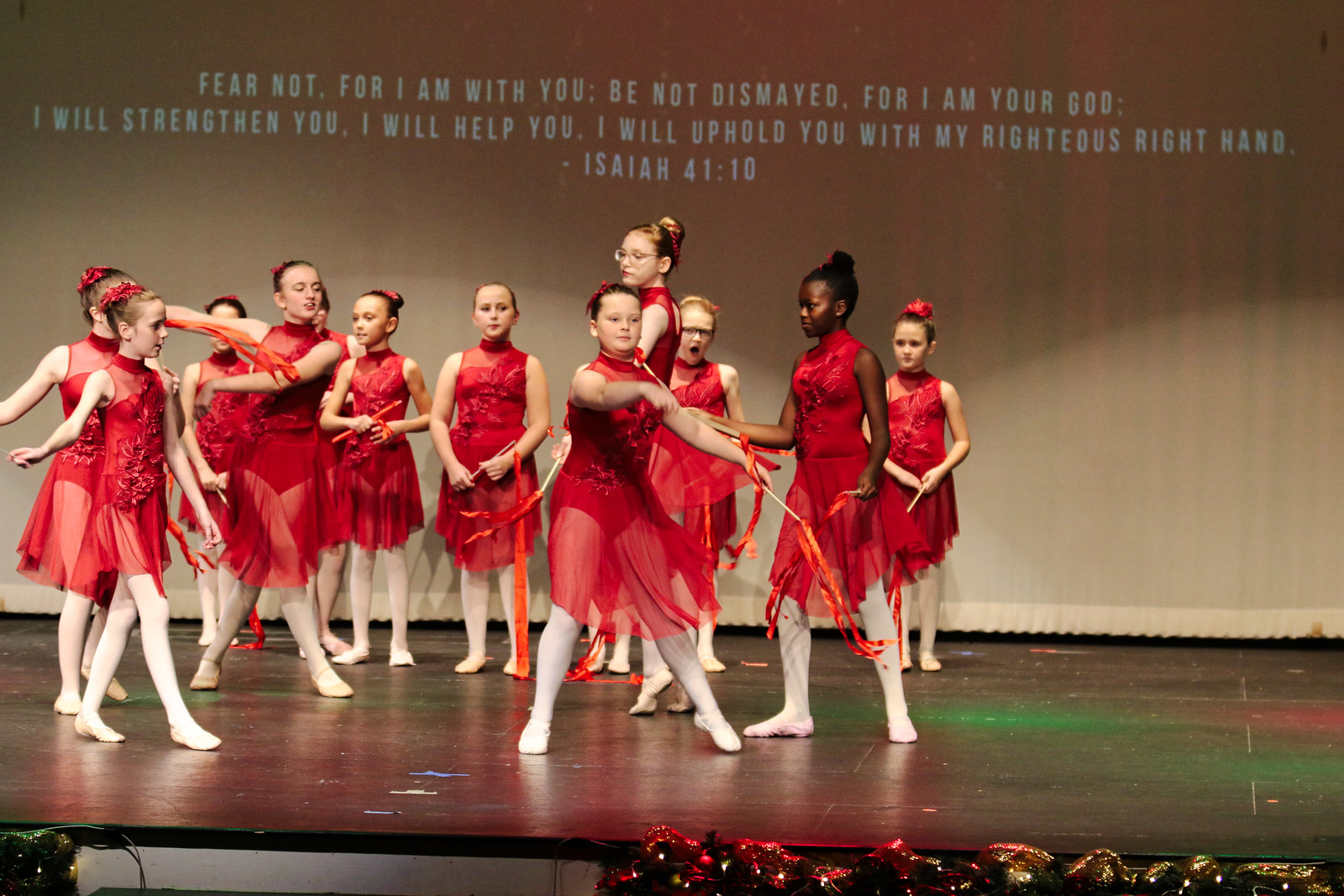The photograph features a group of approximately ten young female dancers performing on an indoor stage, which appears to be adorned with Christmas decorations. The front of the stage is lined with festive embellishments, and there is a visible staircase on the bottom left. Centered predominantly in the image, the dancers are arranged in various ballet poses, some twirling and others standing side by side, holding sticks with red streamers. The girls are uniformly attired in red ballerina costumes, comprising red tutus, lace sleeveless tops, white stockings, and ballet shoes. Their hair is styled in buns adorned with red flowers and decorations. Notably, most of the dancers have white skin except one with black skin, reflecting some diversity. Above them, projected onto the back wall of the stage, is a slide displaying the biblical verse, "Fear not, for I am with you. Be not dismayed, for I am your God. I will strengthen you, I will help you, I will uphold you with my righteous right hand. Isaiah 41:10." The stage is also bathed in red and green lighting, enhancing the holiday theme.